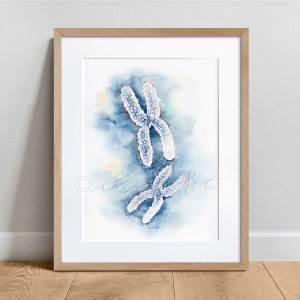This photograph captures a painting leaning against a white wall, above a pale wooden hardwood floor, with a small white baseboard separating the two. The painting, framed in a light brown wooden frame, features a white right-angled mat surrounding the image. The artwork itself is an abstract depiction of two chromosome-like X shapes, slightly curved and positioned vertically with the top X angled to the left and the bottom X angled to the right. These X shapes are a mix of white with blue highlights and are speckled with white dots, set against a backdrop where a blue splotch runs down the center and fades into the white canvas. The blue splotch has a smudging effect around its edges, adding to the abstract quality of the piece. There is an illegible watermark starting with the letter 'K' on top of the bottom X shape.